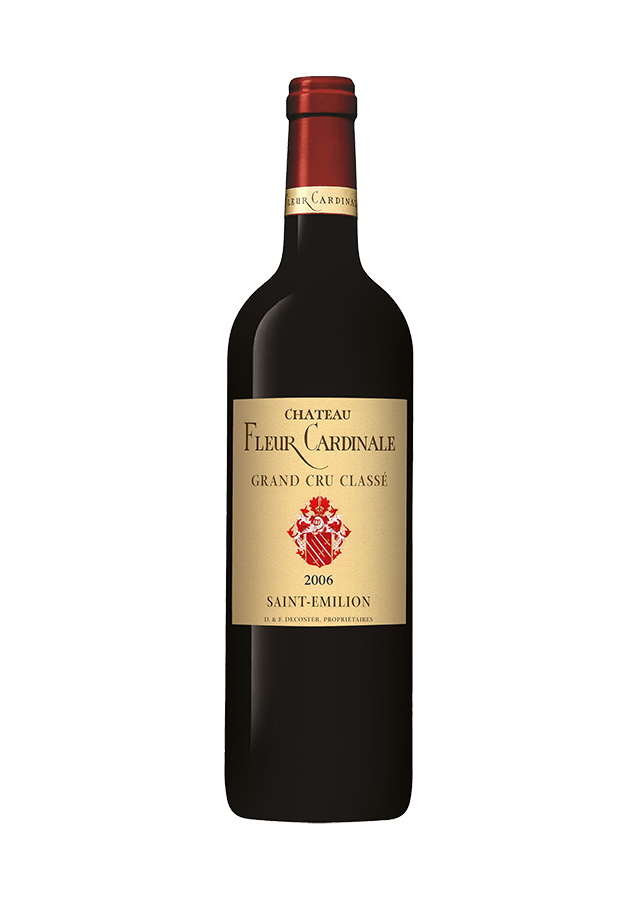The photograph depicts a bottle of French red wine, Chateau Fleur Cardinal Grand Cru Classé 2006 Saint-Emilion, positioned against a stark white background. The bottle itself is dark-colored, almost black, and reflects surrounding light, suggesting a glossy surface. It features a metallic red foil wrap at the top with a thin golden band beneath it. The main label, centered prominently on the bottle, is gold with an ornate red emblem or cross in the middle. The text on the label clearly states "Chateau Fleur Cardinal" with "Grand Cru Classé" written in smaller text beneath it. Below the emblem, the vintage year "2006" is displayed, followed by "Saint-Emilion," indicating the wine's renowned French origin. The overall presentation of the bottle combines elegance with a suggestion of high quality, appropriate for its esteemed pedigree.